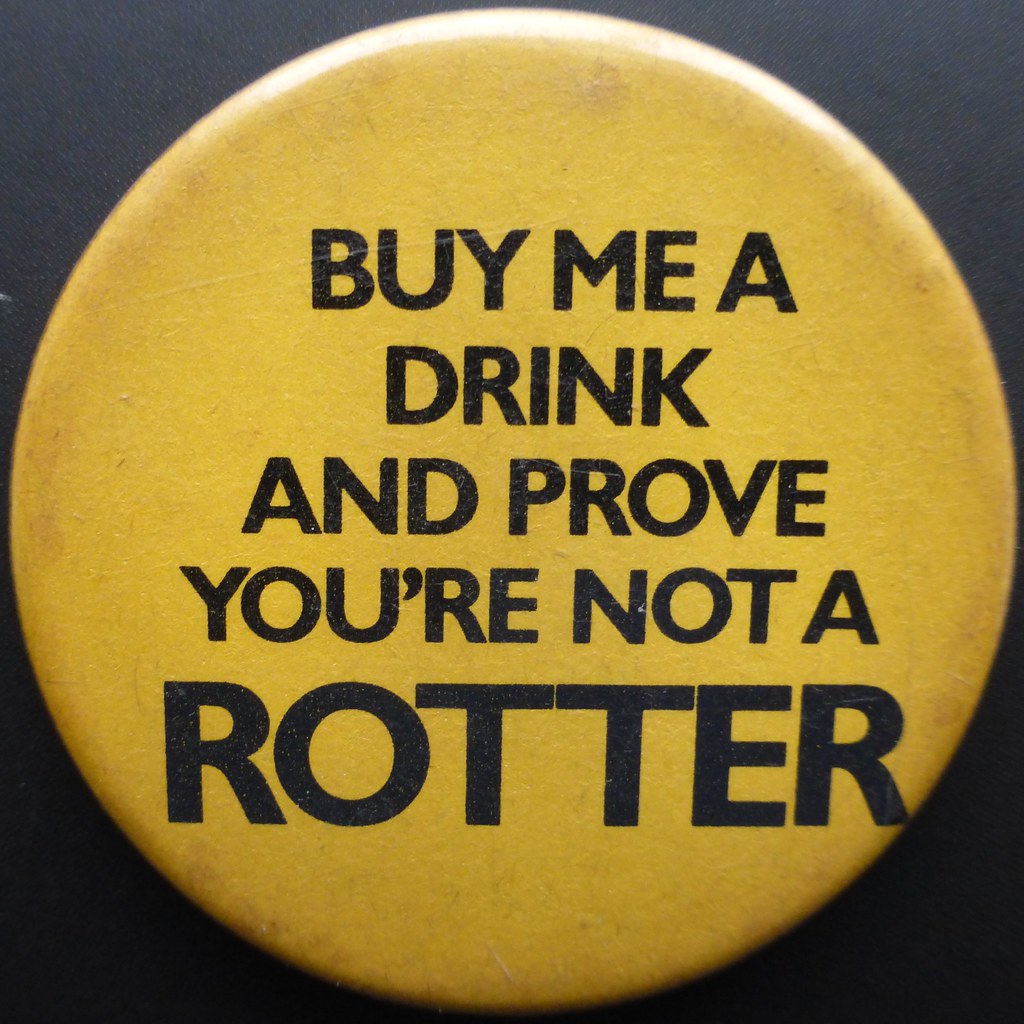The image depicts a worn, round yellow button set against a solid black background. The button appears slightly faded and dirty around the edges, with textures resembling brown and black fibers. In large, bold, black capital letters, the text on the button reads: "BUY ME A DRINK AND PROVE YOU'RE NOT A ROTTER." While most of the text is uniformly sized, the word "ROTTER" stands out with a significantly larger font, so much so that the final "R" spills off the edge of the button. At the top, a white highlight suggests a reflection of light. The entire button dominates the square frame of the image.